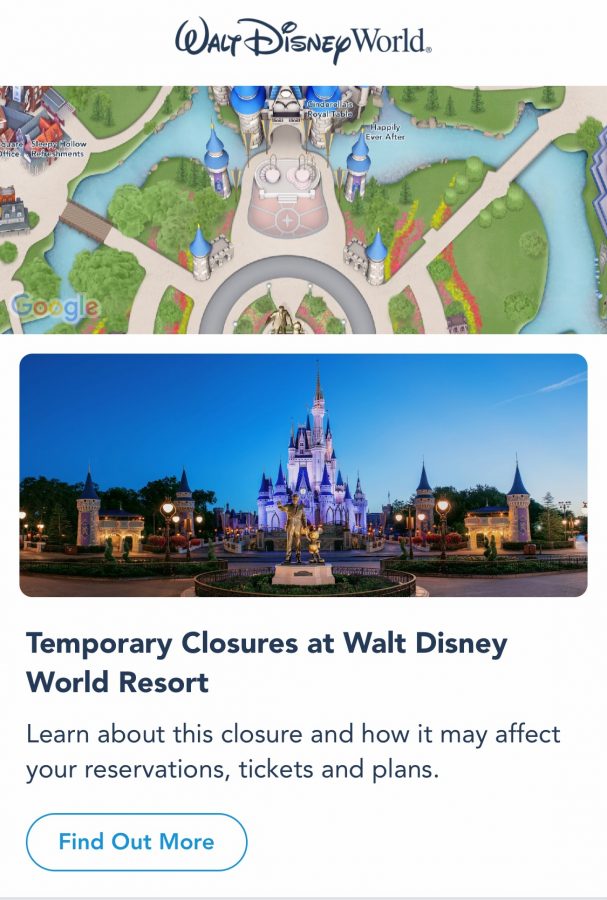The image showcases an overview of Walt Disney World. Prominently placed at the top center is the "Walt Disney World" text, with 'Walt Disney' in the iconic Disney font and 'World' in a regular typeface. Below this text, there is an aerial illustration of the park with a whimsical, cartoon-like appearance.

In the bottom left corner of the illustration, the faint "Google" watermark can be seen. The depicted area resembles an island with a series of small towers, possibly the entrance to the park. Beneath this, a real-life photograph presents a front-facing view of Cinderella's Castle, corresponding to the cartoonish aerial view above.

At the bottom of the image, text reads "Temporary closures at Walt Disney World Resort," followed by information directing viewers to learn about the closures and how these may impact reservations, tickets, and plans.